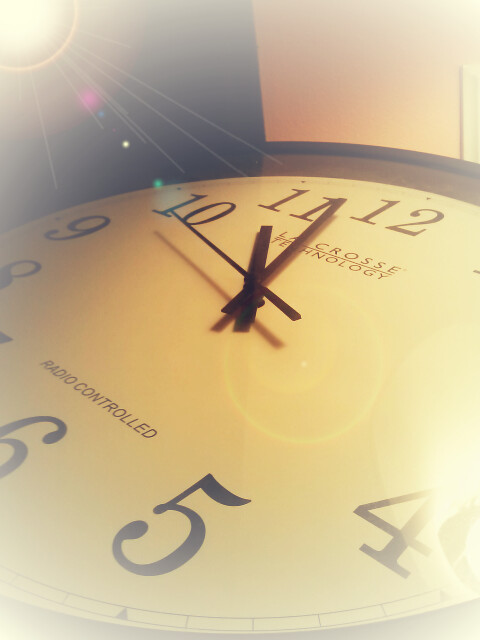This close-up indoor photograph captures a round, Radio Controlled clock with remarkable detail. The image, taken from a very oblique angle at almost a side view, shows the clock lying flat with the perspective from the bottom right corner, looking towards the upper left. At the upper left corner, a yellow sun with rays is visible, casting a light glare onto the clock face, and to the right, a tan wall can be seen. The clock, predominantly occupying the image, features a brown border and a glass cover. The face of the clock is tan, contrasting with the black block-format numerals and black hour, minute, and second hands. The time displayed on the clock is approximately 10:57, with the second hand pointing at the 10. Just below the 12 o'clock position, "LaCrosse Technology" is printed, and above the 6 o'clock is "Radio Controlled." The light source creates a slightly yellowish tinge and a glare on the clock face, adding depth to the photograph.